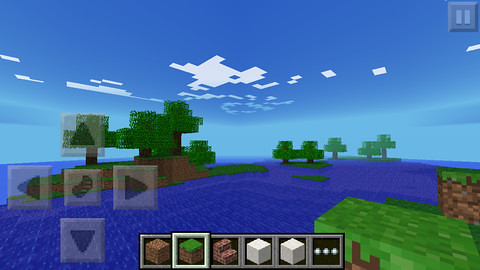This horizontally oriented color screenshot captures a quintessential scene from the game Minecraft. The image depicts a vast, serene blue body of water, interspersed with rectangular, pixelated landmasses covered in green grass blocks. Scattered around the water are a few floating islands, reminiscent of Minecraft's iconic terrain generation. Stalwart, boxy trees dot the landscape, adding to the blocky charm of the environment. Fluffy, pixelated clouds drift across the sky, contributing to the tranquil atmosphere.

In the lower-left corner of the screen, a translucent control overlay featuring directional arrows surrounds a central button adorned with a leaf motif, indicating movement options within the game. Centered at the bottom of the image is a horizontal toolbar housing various tools used for crafting and building. Notably, a silver box highlights the currently selected ground tool within this toolbar.

Additionally, a semi-transparent pause button resides in the top right corner, offering quick access to the game menu. This comprehensive depiction encapsulates the essence of the Minecraft gameplay interface and its distinctive visual style.